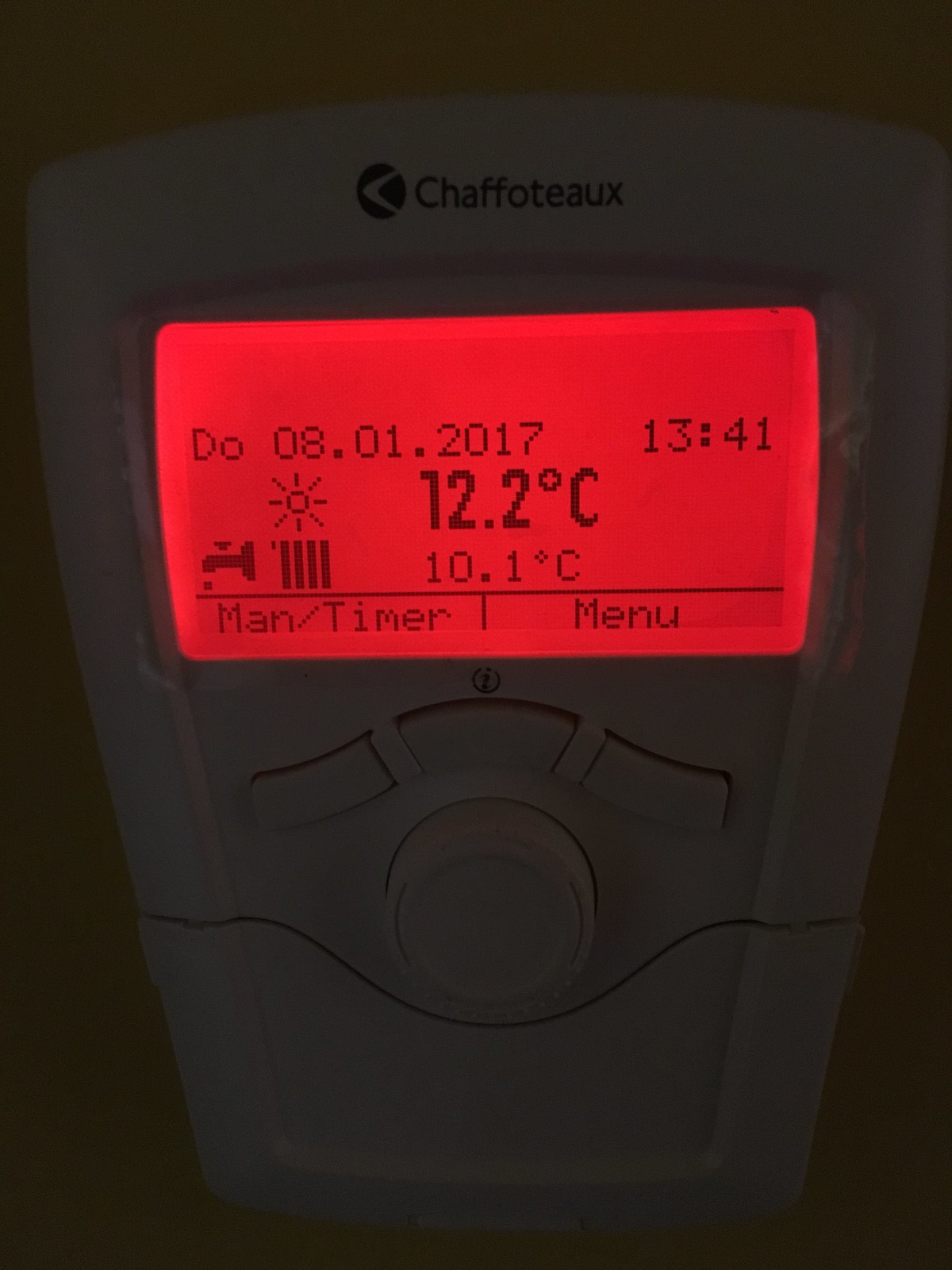This is a detailed close-up image of a thermostat-like device, designed primarily for home use, featuring a sleek, dark-colored body with a white plastic cover. The cover has three buttons situated above a central dial. At the top of the device, there is a red-tinted LED screen, displaying a variety of information. The screen's top left corner reads "DO080.01.2017" in black text, while a timestamp to the right of it shows "13:41". 

In the center of the screen, two temperature readings are shown: “12.2°C” prominently displayed, with “10.1°C” positioned directly below it. The screen also includes various icons, such as a water spigot and a sun above a radiator-like symbol, suggesting functionalities related to heating and water regulation. At the bottom of the screen, a thin black line divides the area into two sections, with "man/timer" on the left and "menu" on the right.

The device's brand name, "Chaffoteaux," is printed in dark letters near the top, accompanied by a distinctive dark logo featuring a white boomerang. Although characterized primarily as a home thermostat, additional icons like the water spigot hint that it may also function as a timer for an irrigation system.